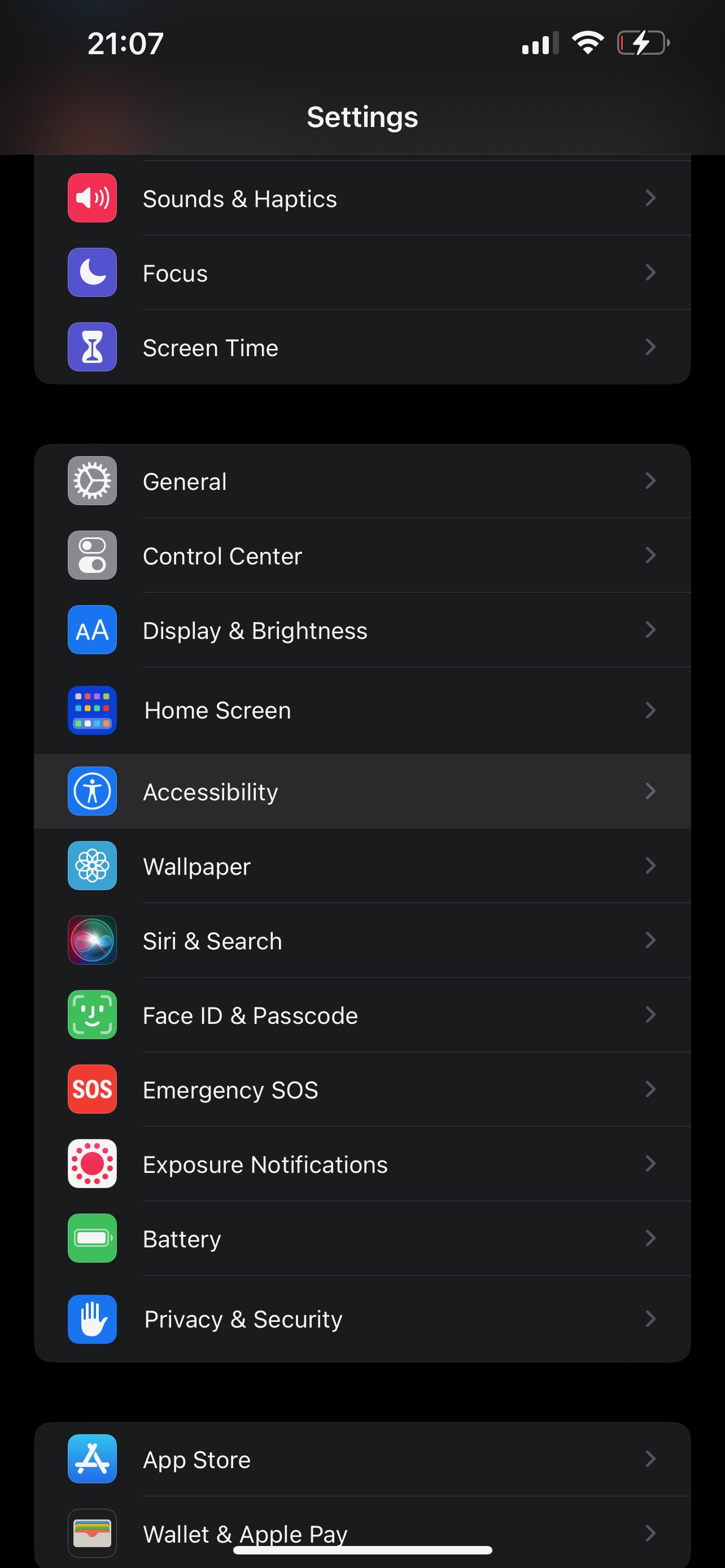The image displays a smartphone screen at 21:07 with three bars of service, a Wi-Fi symbol, and a low battery indicator showing a lightning bolt symbol. The settings menu lists various options including Sounds & Haptics, Focus, Screen Time, General, Control Center, Display & Brightness, Home Screen, Accessibility, Wallpaper, Siri & Search, Face ID & Passcode, Emergency SOS, Exposure Notifications, Battery, Privacy & Security, App Store, Wallet, and Apple Pay.

Additionally, the screen shows several distinct icons:
- A red square 
- A blue square with a moon symbol 
- A blue square with a sand timer symbol
- A gray square featuring settings 
- A gray square containing two round dots inside of ovals
- A blue square with two 'A' letters
- A square filled with various app icons
- A square with a silhouette of a human figure with arms spread inside a circle 
- A light blue circle with a white flower
- A rainbow-colored circle
- A green circle with a face
- A red square with an SOS symbol.

The caption "Spread that" is visible toward the end, seemingly unrelated to the rest of the screen elements. The image reflects a detailed snapshot of a user navigating through various settings and app icons on their device.